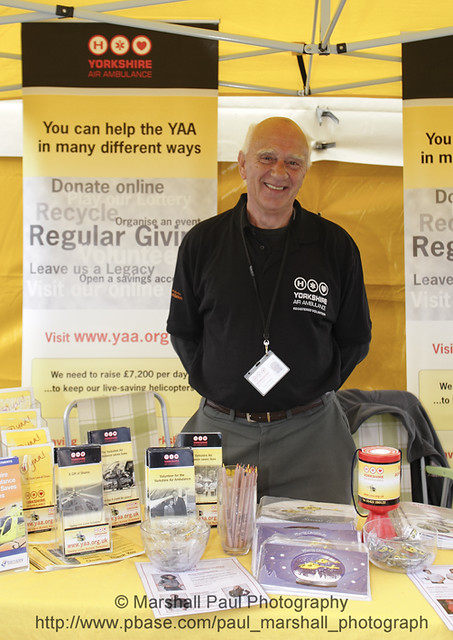The photograph features a bald, elderly man with white hair on the sides, wearing a black shirt with white text on the chest and an identification badge hanging around his neck. He stands just right of center behind a table, with his arms behind his back. The man is dressed in gray pants and a brown belt. The table in front of him is covered with various items, including cardholders with cards, a glass filled with pencils, and informational pamphlets. 

Behind the man, there are two lawn chairs - one to his left and the other to his right, with a jacket draped over the back of the right chair. Flanking him are large banners promoting the Yorkshire Air Ambulance (YAA), with messages such as "Donate Online," "You Can Help the YAA in Many Different Ways," "Recycle," "Organize an Event," "Regular Giving," "Leave a Legacy," and a website URL, www.yaa.org. One banner highlights the need to raise 7,200 pounds daily to maintain their lifesaving helicopter services. The scene appears to be within a tent, under an orange-yellow canopy. At the bottom of the image, there is a copyright notice, "Marshall Paul Photography," with a web address underneath.